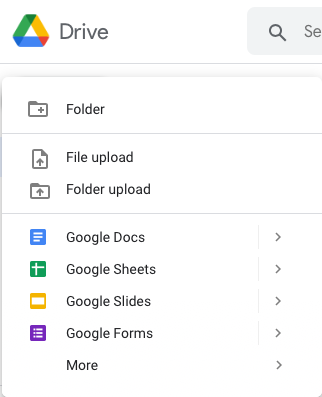Image Caption:

The image is a detailed screenshot of the Google Drive interface, framed in a square with a white background. In the upper left corner, we see the Google Drive logo, featuring a colorful triangle with segments in green, blue, and yellow. The corners of the triangle are darker shades of green, blue, and red. The word "Drive" is written next to the logo.

On the upper right, there's a search bar for easy navigation. Below it, the interface displays various tabs and actions. The first row contains the option labeled "Folder" with a corresponding icon. Below it, another row offers "File Upload" and "Folder Upload" options, each with their own icons.

The interface then moves on to specific Google apps categorized by rows:  

- "Google Docs" is paired with its blue icon.
- "Google Sheets" accompanied by the green icon.
- "Google Slides" next to its orange icon.
- "Google Forms" next to the purple icon, which features white bullet points.

Each of these rows has a small right-pointing arrow at the far right, allowing the user to expand the row to access specific files or create new documents within those categories.